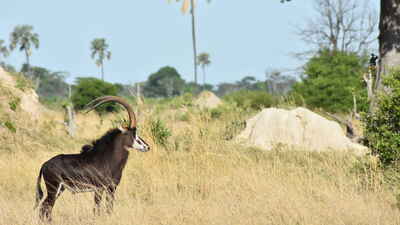The color photograph captures a vibrant outdoor scene in Africa, presented in a landscape orientation focusing on a striking sable antelope. The scene is predominantly dry with golden, yellowish tall grass covering the field. The sable antelope, located in the bottom left corner of the image, stands in profile with its head turned to the right, its slender, blackish-furred back arching gracefully, and long, curved horns extending upward from its head. The antelope's white pointed muzzle, highlighted with distinct black markings, adds contrast to its dark brown body. Surrounding the antelope, a few trees and bushes blend into the background. Dominating the center of the scene is a prominent rock, adding a textured foreground element. Off in the distance, palm trees are visible under a clear blue sky, completing the picturesque African landscape. The photograph embodies a realistic, representational style, capturing the serene yet wild beauty of the natural environment.